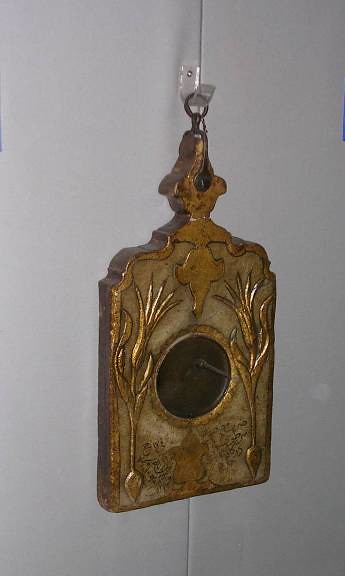A meticulously crafted antique clock, featuring an intricate floral design, hangs elegantly from a plastic hook secured to the wall. The clock boasts a lavish gold finish, accentuating its vintage charm and hinting at its possible metal construction. At its center lies a distinguished brown circular face, complete with a single clock hand affixed to it, adding to its classical allure and timeless aesthetic. The overall craftsmanship and ornate detailing give a glimpse into a bygone era, making it a captivating focal point in any decor.